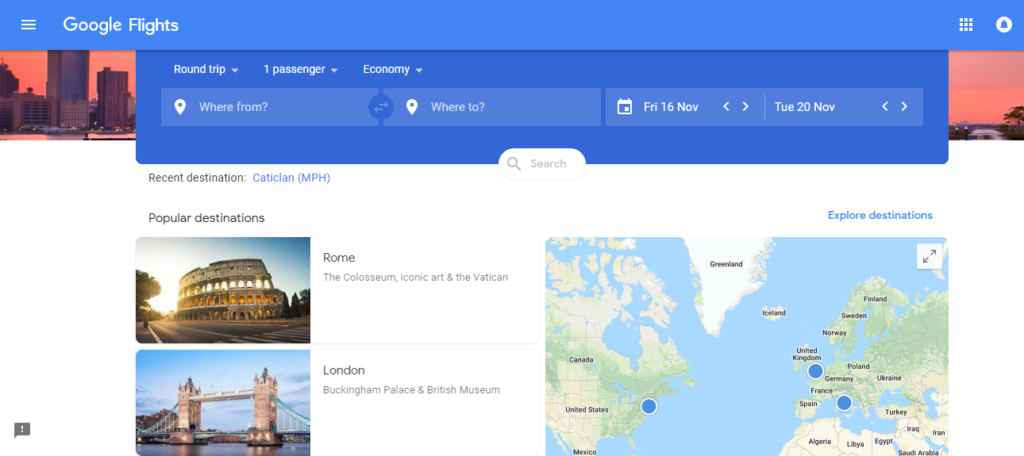The image showcases a screenshot from the Google Flights website. The layout includes a white background on the bottom half of the page, while the top half features a blue bar that spans horizontally across the screen. On the left side of this blue bar, there is a list icon or button. To its right, the text "Google Flights" is prominently displayed in white. Further to the right, there are two additional icons, also in white.

Below the blue bar, an image depicting a city skyline is presented against a reddish-pink background, suggesting a sunset scene. Centrally placed over this image is a blue box displaying flight search information. This box contains options for "Round trip", "1 passenger", and "Economy". Additionally, there are input fields for the departure location ("Where from") and the destination ("To"). Adjacent to these fields are date selectors for choosing departure and return dates for the flight.

Further down, there is a section titled "Recent destination". Beneath it, on the left side, there are popular destination options such as Rome and London. To the right, users can explore more destinations, with a picture of a map serving as a visual aid for this feature.